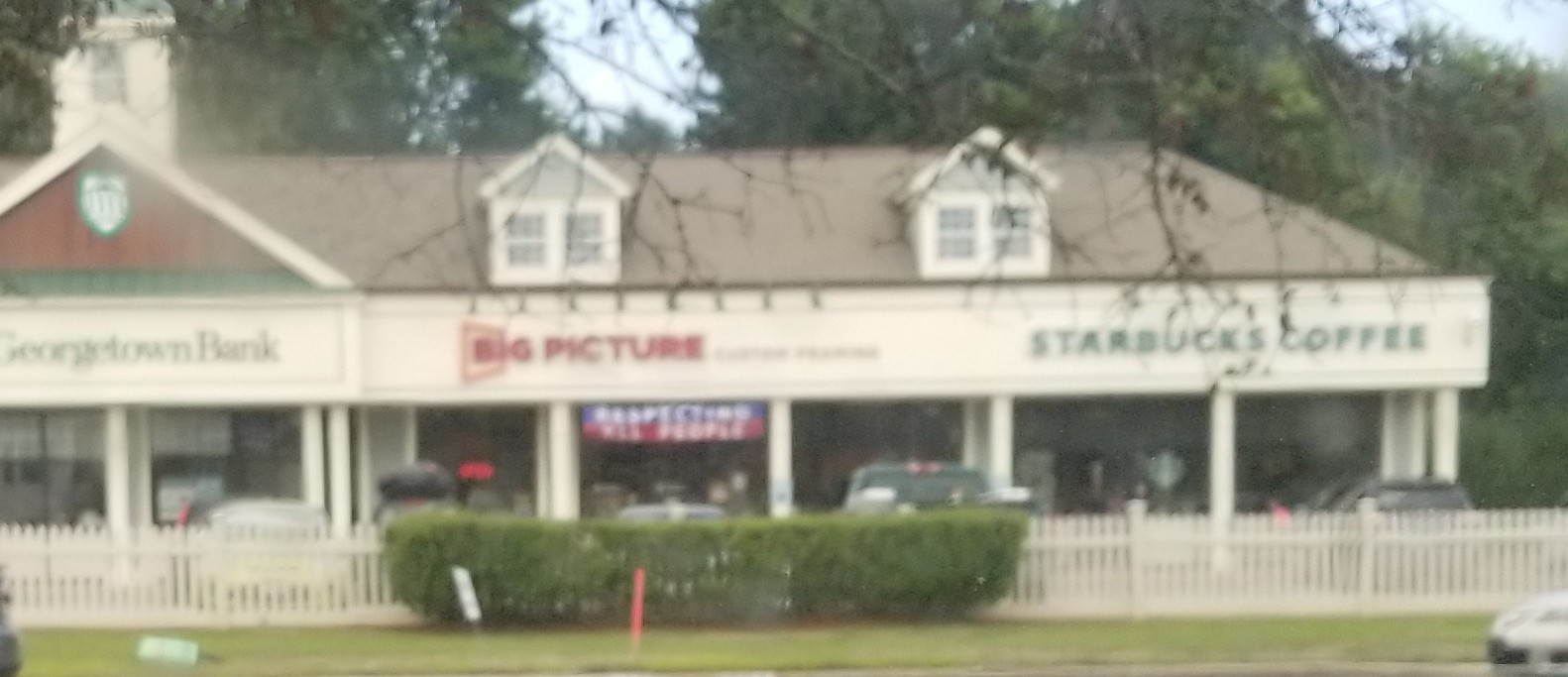This photograph, taken in landscape mode on a sunny summer day, captures a quaint strip mall in a small town. The strip mall features three businesses housed in buildings of a singular design, closely resembling a large house. On the far left is Georgetown Bank, identifiable by its distinct red roof and prominent signage. Just to the right of the bank is an establishment called Big Picture, which features a second-story triangular perch above two small windows, and what appears to be an advertisement below the store name. On the far right is a Starbucks Coffee.

The facade of the strip mall is enhanced by six to seven pillars evenly spaced along its length, and there is a light gray or light tan roof covering the entire structure. In front of the businesses, a white picket fence stretches along the parking lot, with a well-groomed green bush situated precisely in the middle. Several cars are parked in front of the stores, adding to the lively atmosphere. The foreground features a patch of grass and additional landscaped greenery, while the background reveals tall, full trees in various shades of green. The overall effect conveys a charming, well-maintained shopping plaza bathed in pleasant daylight conditions.